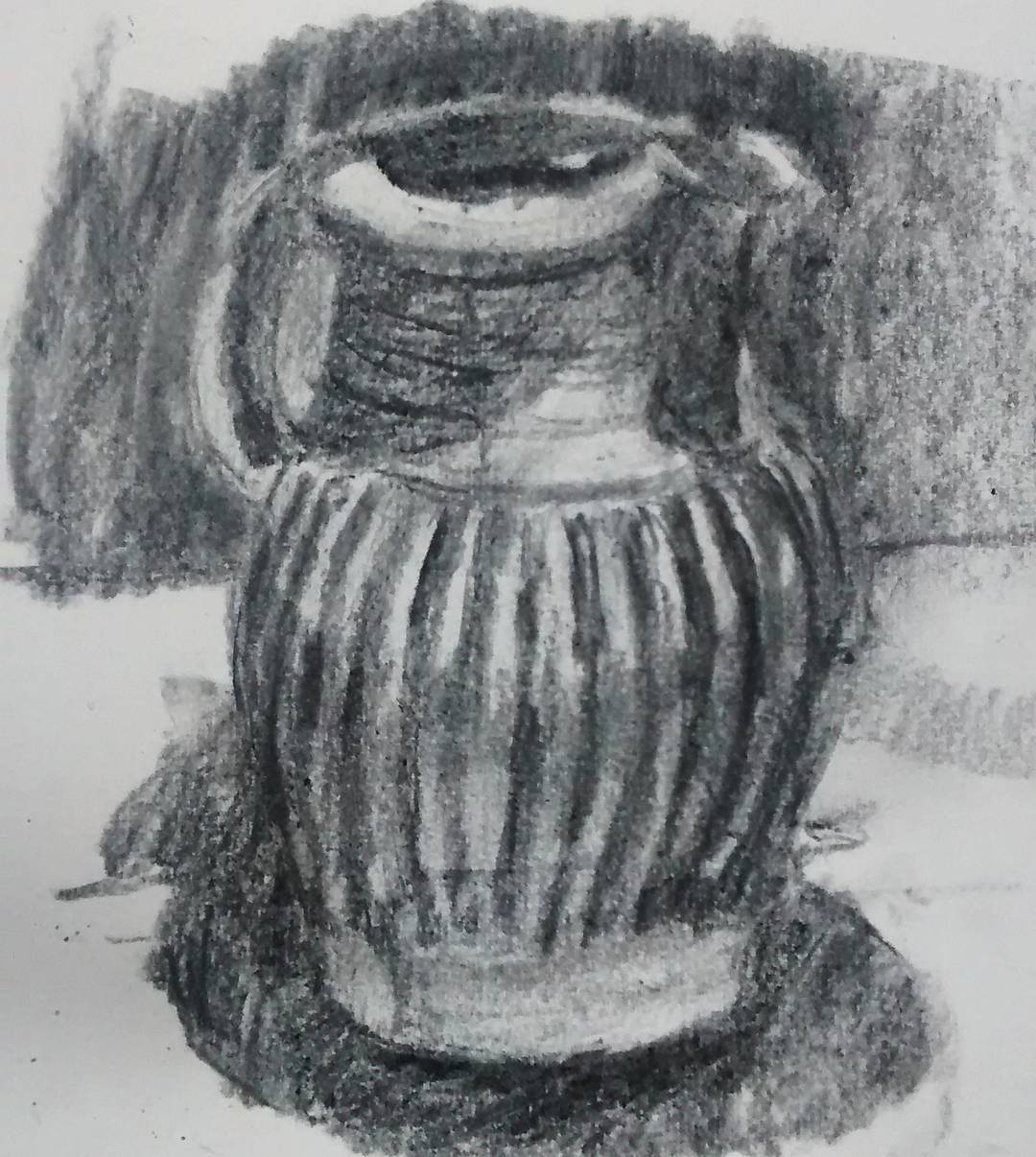The image is a black-and-white drawing, likely done with black crayon or pencil, on a dingy white background. It depicts a vintage water pitcher or urn, characterized by a wide, rounded body with several vertical ridge lines running from top to bottom. The pitcher features a handle at the top on the left side and a singular opening at the top, possibly with a pour spout on the right, though it’s somewhat obscured by the dark shading. The background consists of numerous vertical black lines, adding to the stark contrast against the white table on which the pitcher appears to be sitting. Overall, the artwork has an old and rustic feel, with a significant emphasis on the heavy black shadows cast by the object.